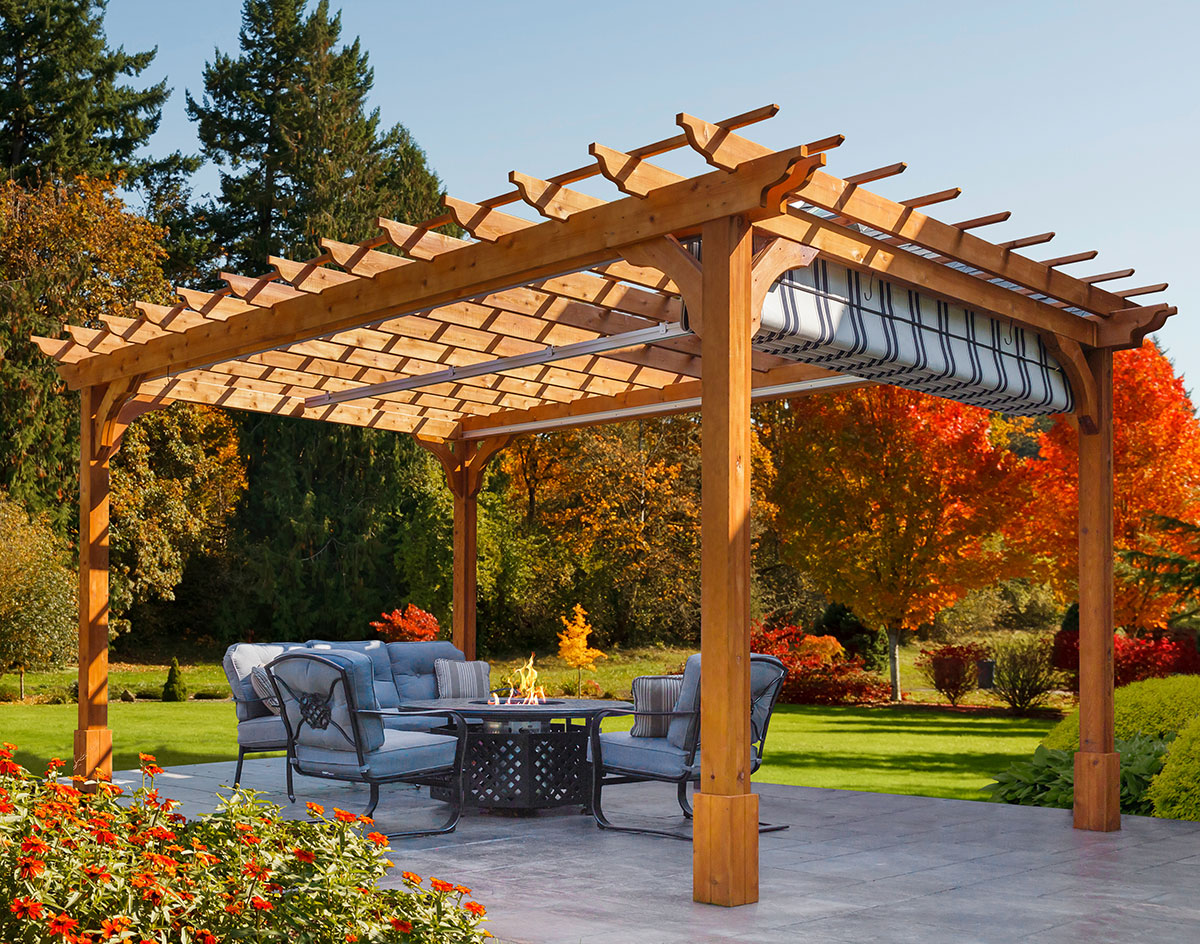This color photograph captures a serene garden scene featuring a pergola in an autumnal setting. The pergola stands on a patio made of gray concrete tiles and is crafted from light brown, redwood-style wood. It includes a black and white screen shade curtain on the right side. Underneath the pergola, a metal-framed fire pit table is surrounded by padded patio furniture, including light blue chairs with gray cushions and a three-section couch. The patio is bordered by vibrant reddish-orange flowers, likely daisies, in the bottom left foreground and green shrubs spilling over its edges.

In the backdrop, a well-tended garden extends with green grass and a variety of trees marking the seasonal transition. To the left, dark green pine trees rise tall, while the background features trees in shades of green transitioning to yellows, oranges, and vivid reds. These deciduous trees highlight the fall season with their colorful leaves. The right side is adorned with more shrubs, completing this picturesque and tranquil park-like yard, perfect for relaxation and gathering.